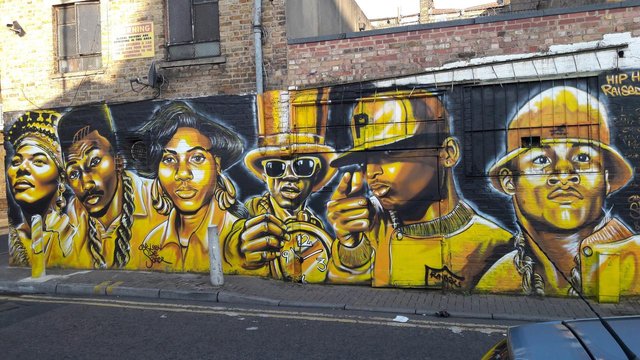This is a color photograph capturing a highly detailed mural on the side of an aged, rough red brick building. The mural, painted in shades of gold and black, portrays six African-American individuals arranged in a row, possibly significant figures in hip-hop culture. In the upper right corner, the text "HIP H RAISED" is prominently displayed.

From left to right, the mural depicts:
1. A woman with an elegant, queen-like headdress, staring pensively into space, possibly Queen Latifah.
2. A man wearing a chain necklace.
3. A woman with curled short black hair and large gold hoop earrings.
4. A man at the center, possibly Flavor Flav, with sunglasses, a large top hat, and his signature giant clock.
5. A man wearing a hat with a 'P' on it, holding his hands in a gun symbol.
6. Another man wearing a yellow hat, with features glazed in a golden hue.

The scene includes part of the street and the sidewalk in front of the mural, with the hood of a car just visible in the lower right corner. Each portrait is detailed with gold accents and set against a deep black background, creating a striking visual contrast against the rough brickwork.